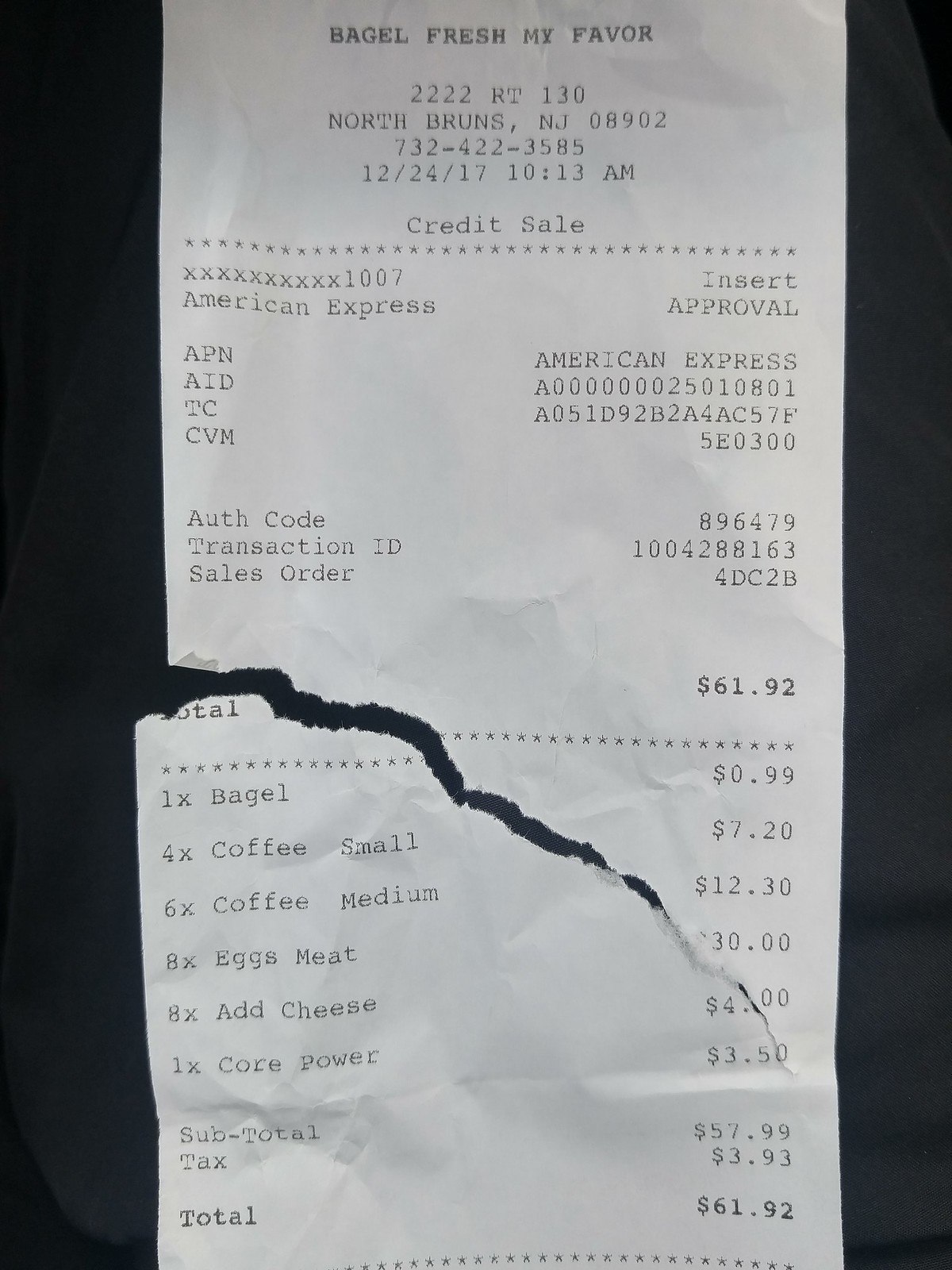This detailed caption describes an image of a torn receipt from North Brunswick, New Jersey, dated New Year's Eve of 2017 at 10:13:18 a.m. The transaction was completed using an American Express credit card. The purchase includes a variety of items: one bagel, four small coffees, six medium coffees, and eight servings of eggs with meat. Notably, eight servings of eggs with cheese were ordered, with some explicitly without cheese. Additionally, there is an item listed as "one quart power," though the specific item is unclear. The total amount paid for these items is $61.92, while the subtotal for the purchase is $57.39, suggesting the inclusion of tax or additional fees to reach the final amount. The receipt, printed on white paper that has faded to gray, is nearly torn in half and placed against a black background for the photograph.